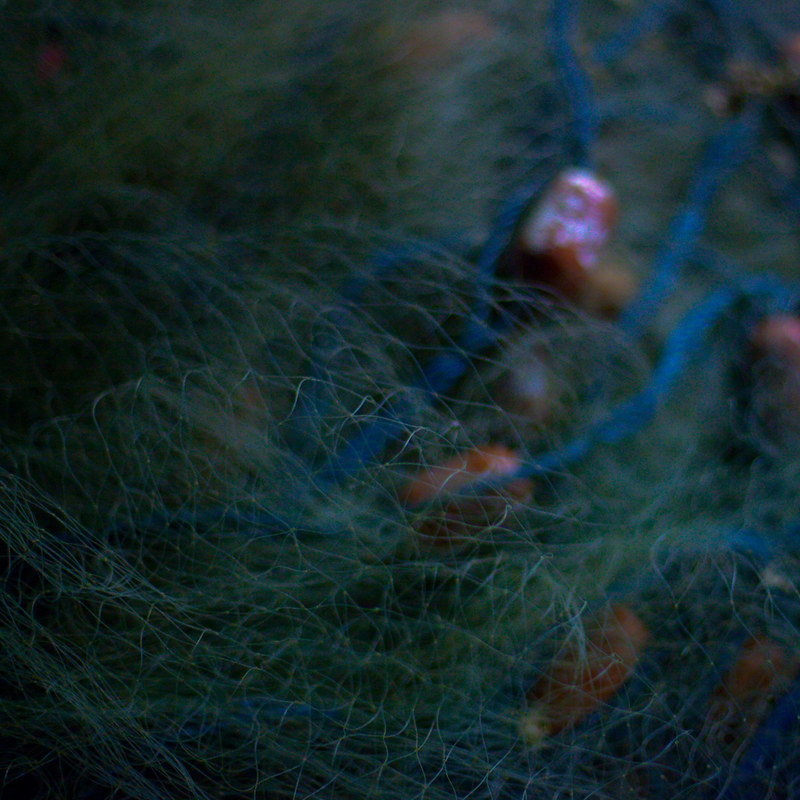This is a color photograph, approximately six inches by six inches, which captures a tangled bundle of fish netting. The main focus of the shot is the net itself, characterized by thicker blue strands outlining fine green mesh. Despite the close-up, the image is quite out of focus, making it challenging to discern the surroundings or whether the location is indoors or outdoors. Scattered within the net are small, shiny orange objects, possibly buoys, with one notably reflective item featuring white spots. The net's texture and the jumbled mesh dominate the entire frame, while all corners, especially the upper left, are considerably darker, adding to the overall blurred and indistinct appearance of the photo.